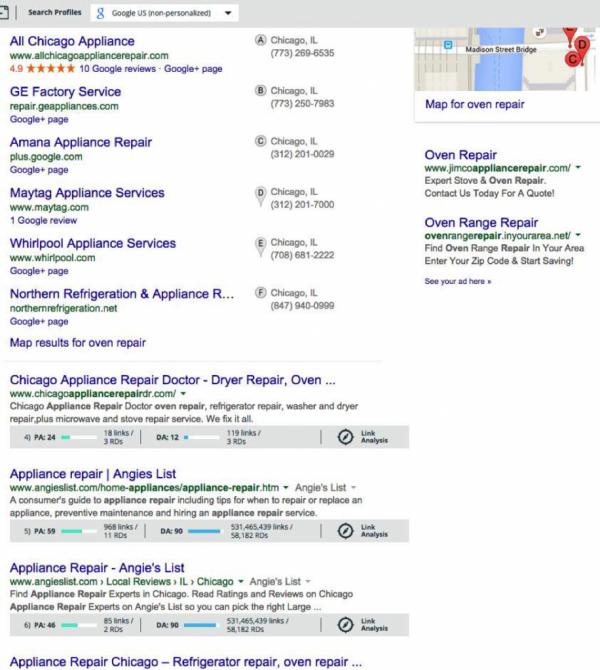The provided image showcases the results of a Google search for "Oven Repair." In the upper right-hand corner, there is a detailed map labeled "Map for Oven Repair," listing several appliance repair services along with three noted fines. The businesses displayed include:

1. All Chicago Appliance
2. GE Factory Service
3. Amana Appliance Repair
4. Maytag Appliance Repair
5. Whirlpool Appliance Services
6. Northern Refrigerator and Appliances

Adjacent to the map, there are additional search results titled "Oven Repair" and "Oven Range Repair." Below this section, further listings appear, such as:

- Chicago Appliance Repair Doctor, which also offers services for dryers and ovens (additional details are truncated by ellipses).
- Appliance Repair Angie's List, which is mentioned twice.

The three listings at the bottom of the search results provide more comprehensive information about their services.